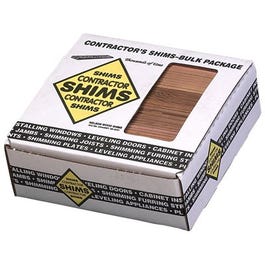This image depicts a white cardboard box containing wood shims, labeled as a "Contractor's Shims Bulk Package." The box features a square top and bottom with narrow rectangular sides. Prominently displayed at the top in bold black print are the words "Contractor's Shims Bulk Package." Below this text, a yellow diamond-shaped logo repeats the phrase "Shims, Contractor Shims, Contractor Shims." There is a small plastic window on the top and an oblong hole through which the brown, wood-colored shims are visible. Black horizontal bands stretch across this window. Surrounding the edges of the box is a black banner embellished with white text that is difficult to read. However, within these black sections, detailed purposes for the shims are listed, including "Installing Windows, Leveling Doors, Cabinet Install, Door Jams, Shimming Joists, Shimming Plates, Leveling Appliances." This informational text is also found on the sides of the box, accompanied by another yellow diamond-shaped logo identical to the one on the top.